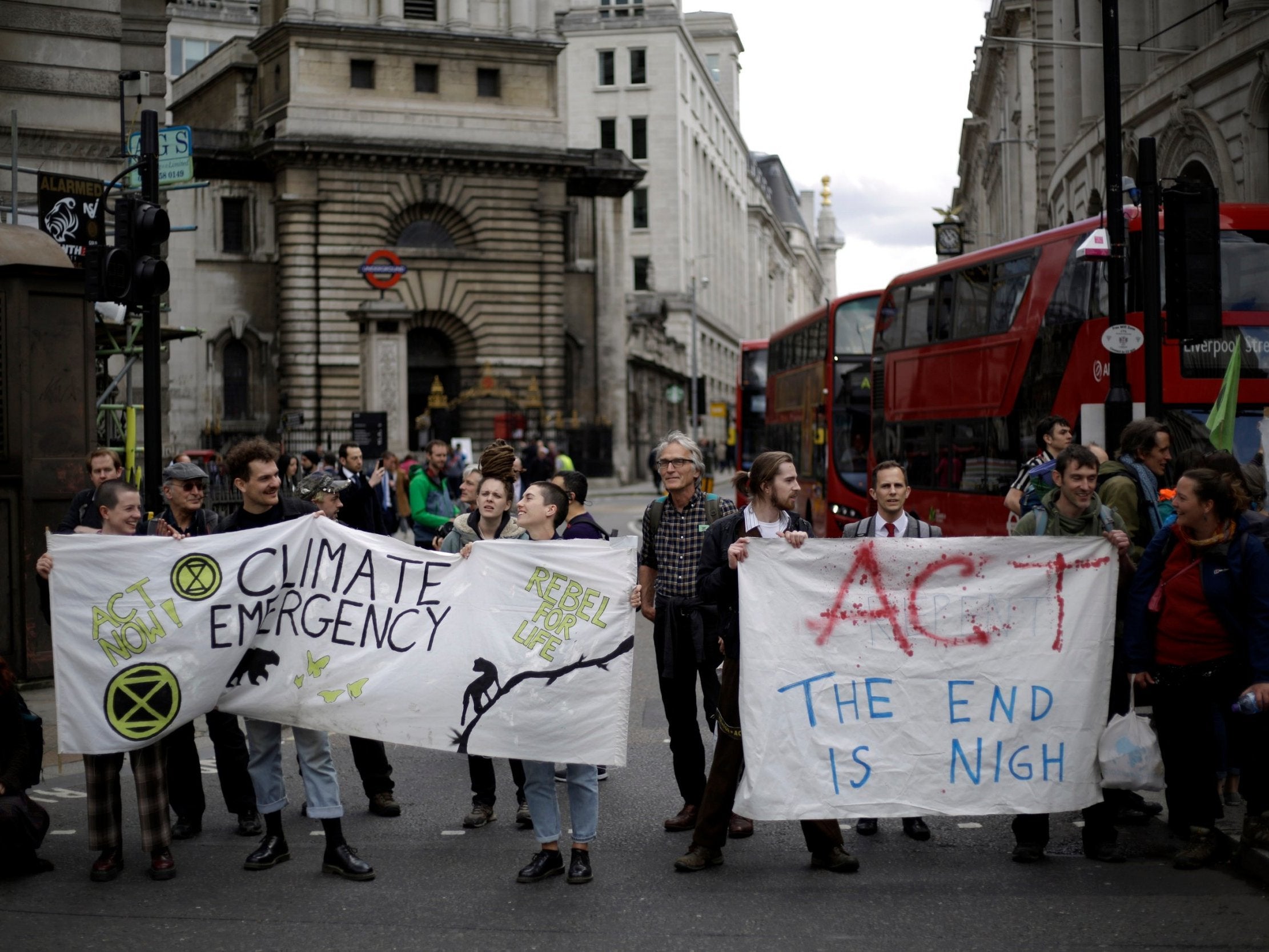This photograph captures a candid protest scene on a dreary day in London, with the iconic red double-decker buses marked "Liverpool Street" visible in the background. The protest centers around climate action, with two prominent signs held by the demonstrators. 

The first protest sign, a long horizontal banner held by three people, declares "Act Now" in green, "Climate Emergency" in black, and "Rebel for Life" in green. It also features hand-drawn illustrations of a bear, butterflies, and a tree branch, all detailed in black and green. The second sign, held by two men looking at each other, reads "Act" in red and "The End is Nigh" in blue. 

The group appears in good spirits, with participants smiling and engaging with one another. The background shows tall, gray stone buildings and a bustling street, with people going about their everyday lives, dressed mostly in business casual attire. This evocative image emphasizes both the urgency and communal spirit of the climate emergency protest.